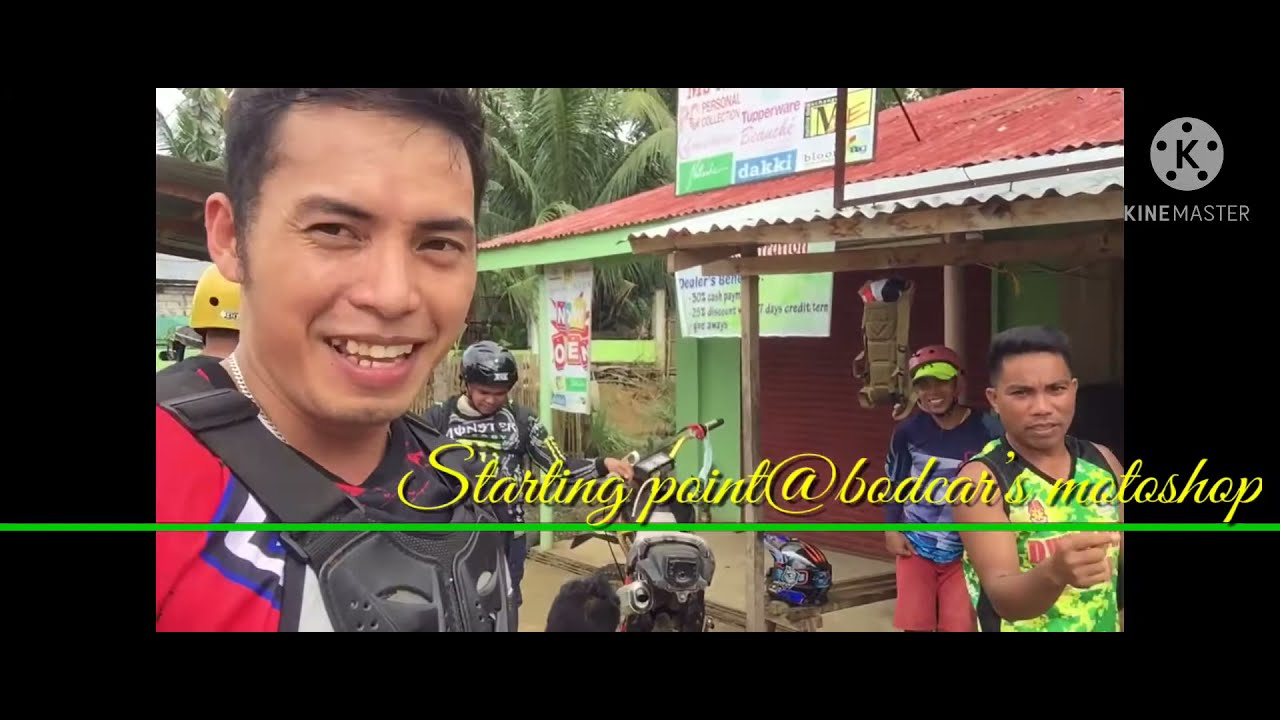The photograph captures a vibrant scene in front of a shop named "Starling Point at Baccarat's Moto Shop," marked by yellow cursive text overlaid at the top, underlined by a green line stretching the width of the image. The setting is tropical, evidenced by palm trees visible in the background. The central figure on the left is a smiling, dark-haired man of Asian descent, wearing a red shirt and a type of plastic vest resembling body armor, accompanied by a silver chain. He appears to be engaging with the camera as if talking. Surrounding him are four other men, each uniquely outfitted: one in a green shirt, another in a blue shirt with red pants, and two others sporting helmets. One helmet is yellow, worn with a black shirt, while the other is black, paired with a matching shirt. The latter is depicted touching a moped positioned centrally in the image. They stand in front of a small building with a red garage door and a corrugated metal roof, suggesting a long history of changes. Additional signage, some unreadable due to language and size, adorns the shop. This lively scene suggests a group poised for an adventure, possibly a bike race or a day of riding mopeds.